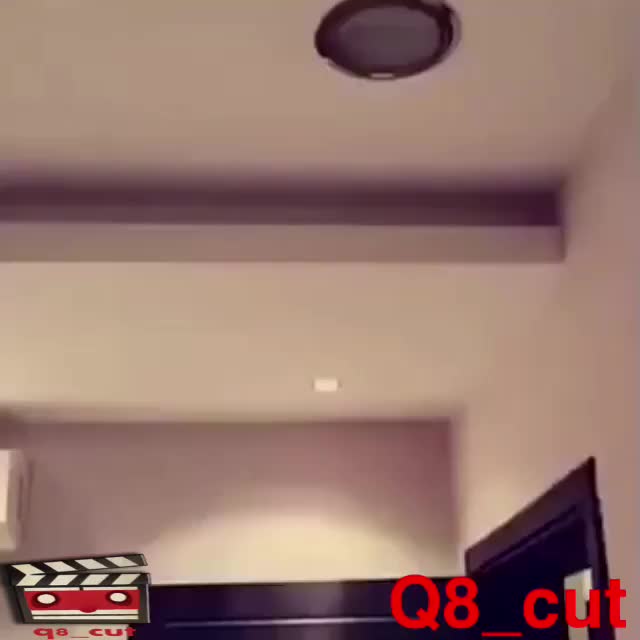This image captures the interior of what appears to be a small office room, focused primarily on the ceiling. The ceiling features a recessed section with a round light fixture characterized by a black outer rim and a gray filling, though the light is not illuminated. The walls are predominantly white, with dark trim around a door frame that partially enters the frame. A dark brown or possibly black door with matching trim is visible below the ceiling.

Additionally, there's a white object affixed to the left side of the wall, likely an air conditioning unit. Prominently in the lower corners of the photograph are two identical text elements: a cartoon-like movie clapperboard rendered in black, white, and red in the lower left-hand corner, and in the lower right-hand corner, larger orange type that reads "Q8_cut." Both display the text "Q8_cut," though the exact color differs slightly between the two instances.